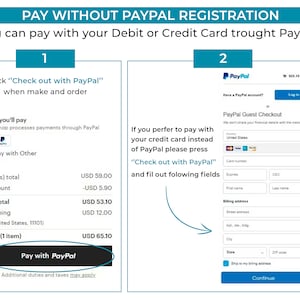The image features a seemingly deceptive email message with various elements and text instructions. At the top, there is a light blue banner with white text stating, "Pay Without PayPal Registration." Below this, a section with a white background contains the message, "You can pay with your debit or credit card through PayPal," with a noticeable misspelling of "through" as "trought." 

The layout includes two prominently numbered blue boxes. Box number one advises, "Check out with PayPal when making an order," and below this instruction, there are multiple charges listed. A black rectangular box circled in blue, labeled "Pay with PayPal," is positioned under these charges.

On the right side of the image, blue box number two instructs, "If you prefer to pay with your credit card instead of PayPal, please press 'Check out with PayPal' and fill out the following fields." Adjacent to this, there are various sections designed for inputting personal information. The overall presentation and incorrect spelling contribute to the impression that this might be a scam email designed to mislead users.